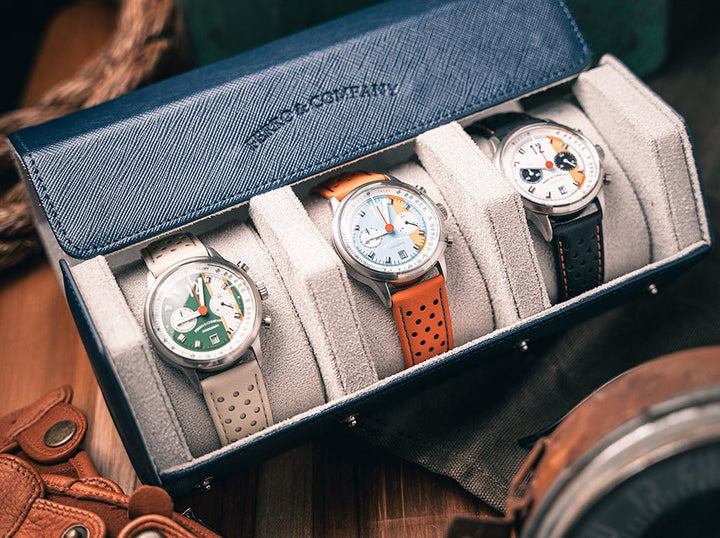This indoor, artificially lit, square photograph showcases a staged display of three watches inside a blue, stitched display box labeled "Farrell and Company," which is difficult to completely read. The box's interior is white, fitted with cylindrical holders divided for each watch. The first watch features a white band with a green face; the middle has an orange band with a light blue face; and the third flaunts a black band with a white face accented with navy blue. The box is slightly angled downward to the left and rests on a wooden tabletop. Surrounding the box, the lower left corner reveals some brown leather with snaps, the lower right corner displays a vague silver and rusty circular object, and the upper left corner hints at a piece of thick, heavy rope. The entire scene includes various accessories that are hard to identify clearly.